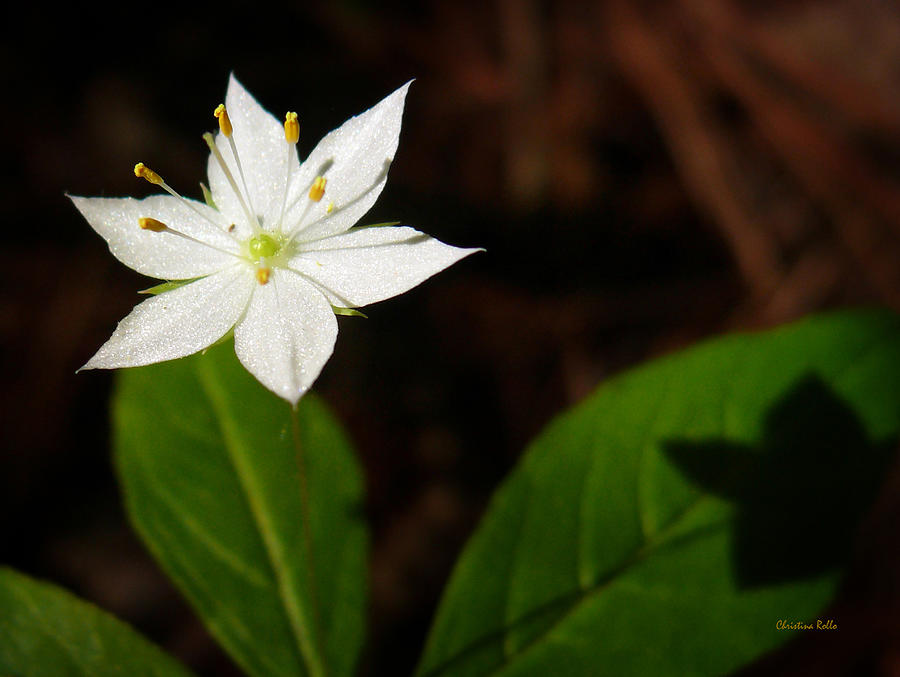This image captures a close-up view of nature, focusing on a single white flower with six shimmery petals, located prominently in the top left corner. The flower features a spherical, light green center from which several white stems protrude, each tipped with yellow pollen pods. Surrounding the flower, large, leafy green leaves occupy the bottom of the image, with three leaves predominantly visible—two of which stand out more clearly than the partially obscured one on the left. The background of the image is dark, with indistinct shades of brown smudging particularly in the top right area. The only text present is the cursive yellow signature "Christina Rojo" at the bottom right, indicating the artist. The natural setting and rich palette of brown, white, yellow, green, and orange hues suggest this scene could be from a garden or wilderness area.